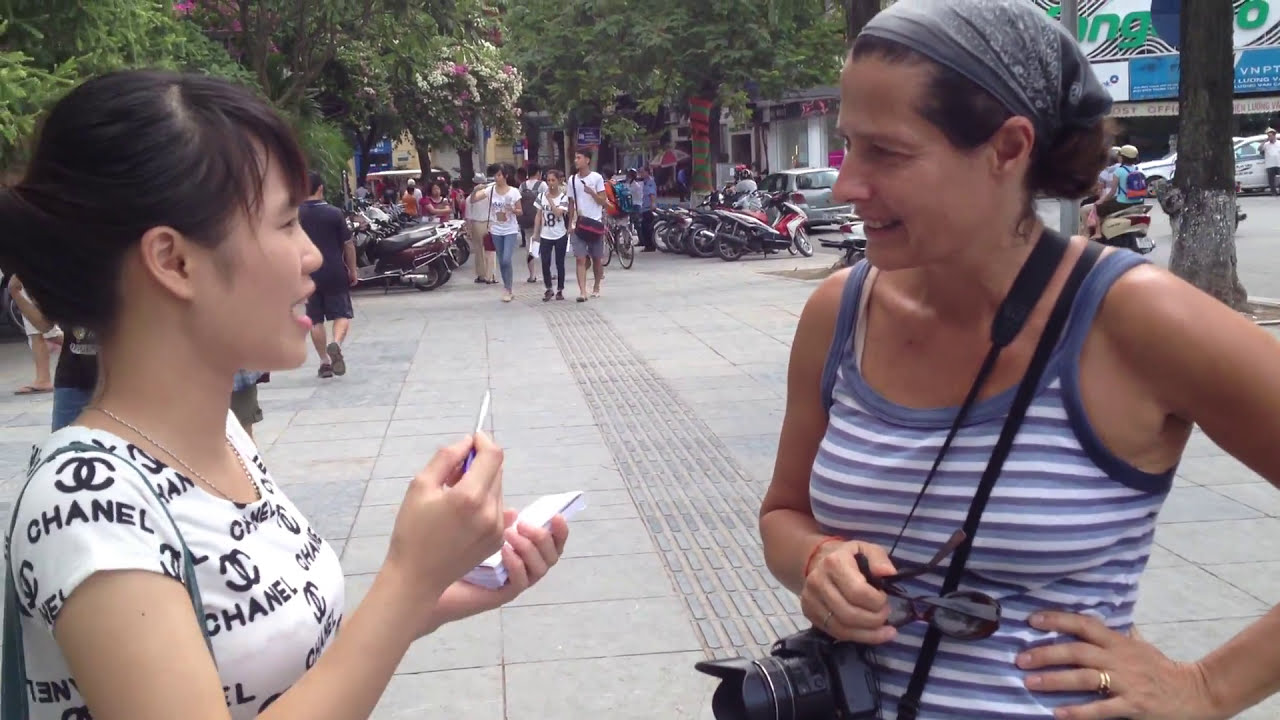In the image, two women are engaged in a conversation in what appears to be a large, cemented area, possibly a spacious patio. The woman on the left, who has Asian features, is dressed in a chic white and black Chanel shirt adorned with the brand's emblem. She holds a notepad and a pen, indicating she might be taking notes. The woman on the right is slightly taller, sporting a blue bandana and a casual blue and white striped tank top. She has a camera hanging around her neck and is holding a pair of sunglasses. They are surrounded by a bustling background featuring trees, unidentified shops, and a few people walking towards them. Additionally, there is a line of parked scooters and motorbikes, adding to the urban setting. The palette of the scene includes an array of colors such as white, blue, black, gray, green, pink, and red, providing a vibrant context to their interaction.